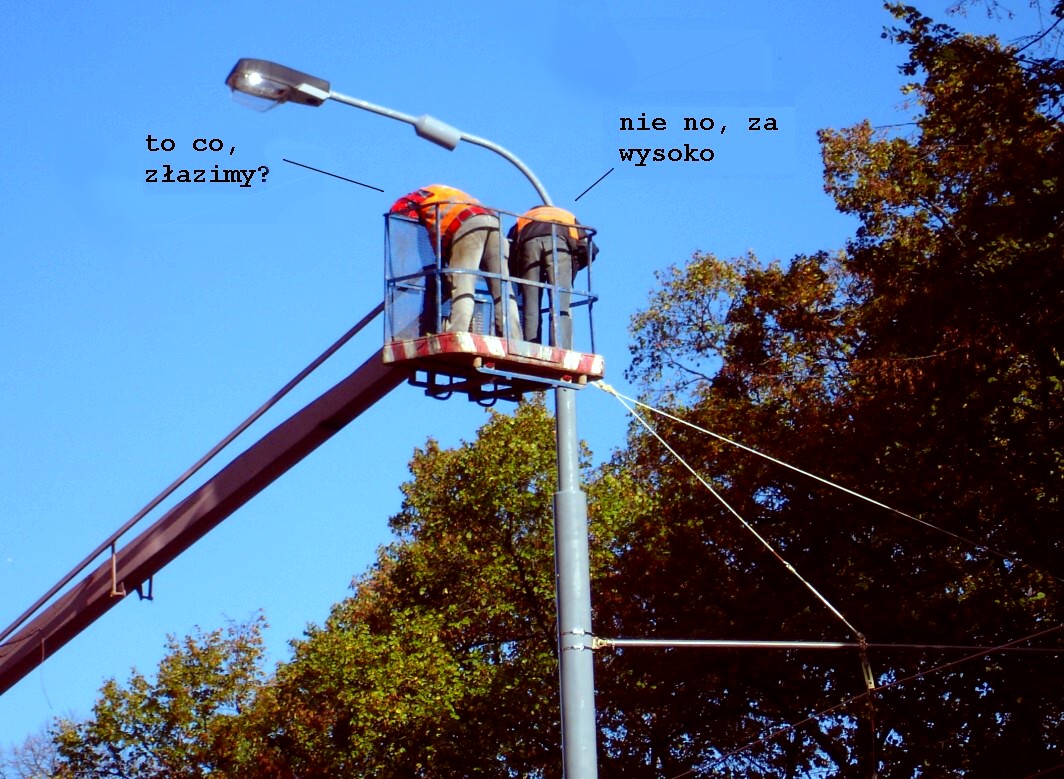A brightly colored outdoor photograph captures a vibrant medium-toned blue sky above a line of tall trees, some still lush green while others are transitioning to reds and browns. Dominating the center of the image, a silver pole with a street lamp arches leftward with its light directed downward. Attached to the pole are guy wires extending off to the right. Below the lamp hangs a blue metal and mesh bucket from a cherry picker, secured with red and white safety stripes. The bucket's arm, a large metallic red beam, reaches up from a truck that is out of the frame. Inside the bucket are two workers, one in gray pants and the other in blue jeans, both wearing bright orange safety vests. They bend forward, peering over the bucket's edge. Above them, in superimposed black text, are two lines of communication in Polish, hinting at a dialogue between the men. The left line reads "TO CO, ZŁAZIMY?" while the right one responds, "NIE NO, ZA WYSOKO." The photograph, though somewhat unfocused and with unusually bright colors as if reproduced many times, radiates a vividness that amplifies the scene's dynamic energy.